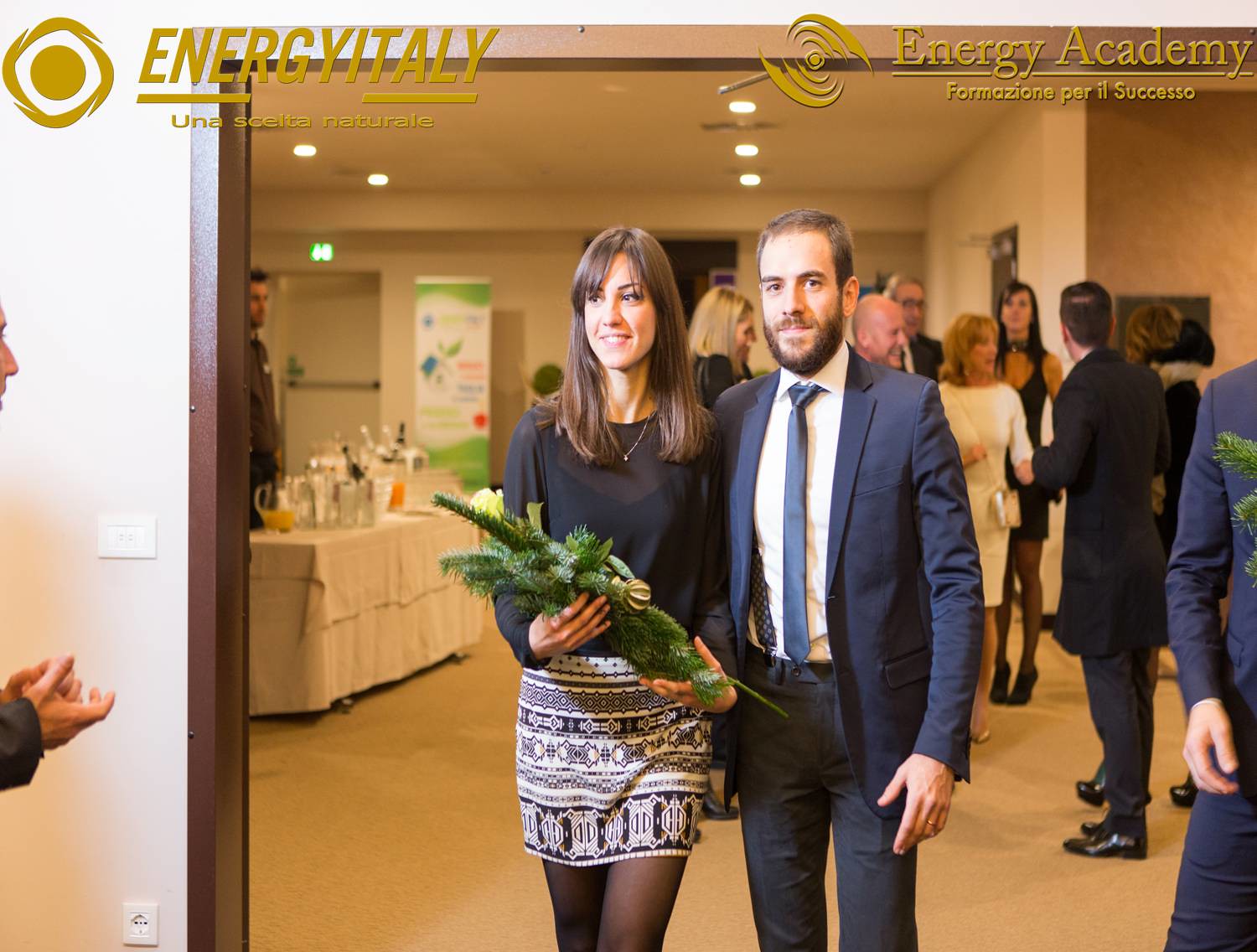In the image, a well-dressed couple is prominently walking through what appears to be a festive banquet hall, likely around Christmas time due to the woman holding a decorative fir sprig adorned with ribbons. The woman on the left has shoulder-length dark brunette hair with bangs and wears a black top paired with a black and white patterned skirt and black tights. She smiles as she glances leftward. The man beside her has short brown hair, a brown beard, and wears a coordinated blue suit, blue tie, white shirt, and printed suspenders. Both are facing the camera, and the man's hands rest at his waist.

Behind the couple, several people dressed formally in suits and dresses are gathered, conversing and mingling. Notably, one person appears to be clapping, possibly indicating a celebratory moment for the couple, like an engagement or wedding. 

Against the beige walls in the back, double exit doors are visible, along with a banquet table covered with a white tablecloth set up with drinks and attended by a server. Logos reading "Energi Italy" and "Energi Academy," along with additional text and circular designs in gold, adorn the top left and right corners of the room, rounding out the details of this festive and elegant setting.